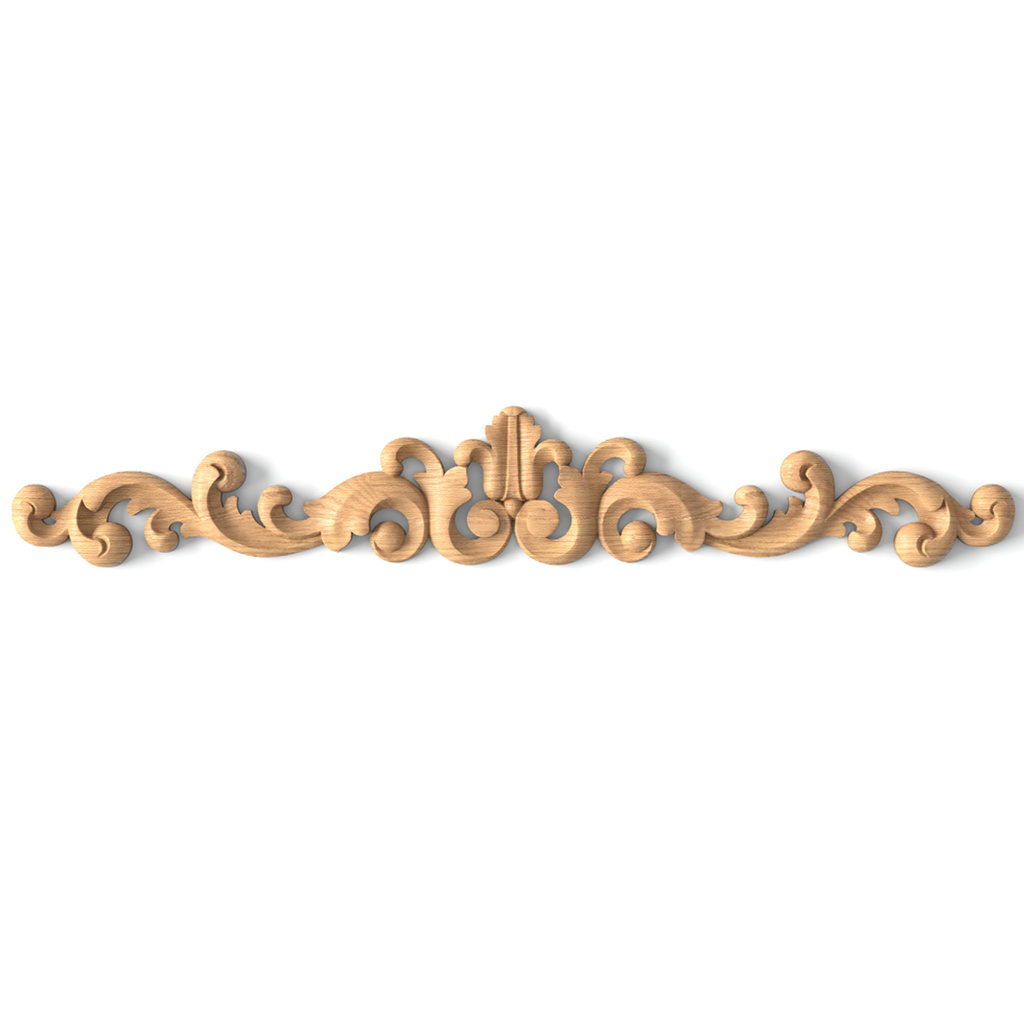The image depicts an ornate wooden filigree carving, intricately designed with a light brown hue and fine dark grains. This elongated piece features symmetrical swirling details and leaf-like patterns, with each side mirroring the other. At the very center is a focal design resembling a fleur-de-lis or tulip, with curving patterns radiating outward like waves or gusts of wind. Set against a white background, the carving casts a shadow to the right, indicating a light source from the left. This elegant piece resembles a decorative panel that could be used to adorn the top edge of a mirror, a door frame, or a mantelpiece, adding a vintage, high-class touch.